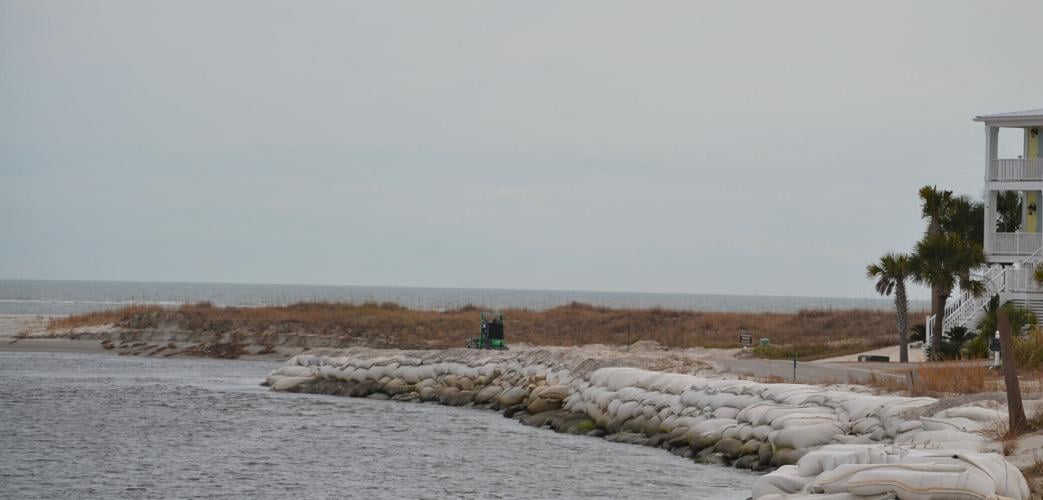The outdoor image captures a very cloudy day near a rocky waterfront, with heavy overcast skies creating a blanket of medium gray. The scene is likely from a coastal region, suggesting a beach-like environment with gray, lightly undulating ocean waves. Dominating the left side of the picture is the expansive gray ocean water and a shore lined with overlapping rocks or possibly sandbags, serving perhaps as a barrier against tides or storms.

In the middle of the image, patches of brown grass hint at an untended portion of land. To the far right, partially visible, stands a three-story white house, elevated with stairs leading to its main floor. Three large palm trees are positioned in front of the house, adding to the ambiguity of the location—potentially somewhere in the south. The house is fronted by a winding street that curves into the background, where a sign is faintly visible against the gray, horizon-blurred scenery.

Amidst this coastal tableau, a lone individual appears to be riding a mower, contributing a touch of human activity to the otherwise static scene.